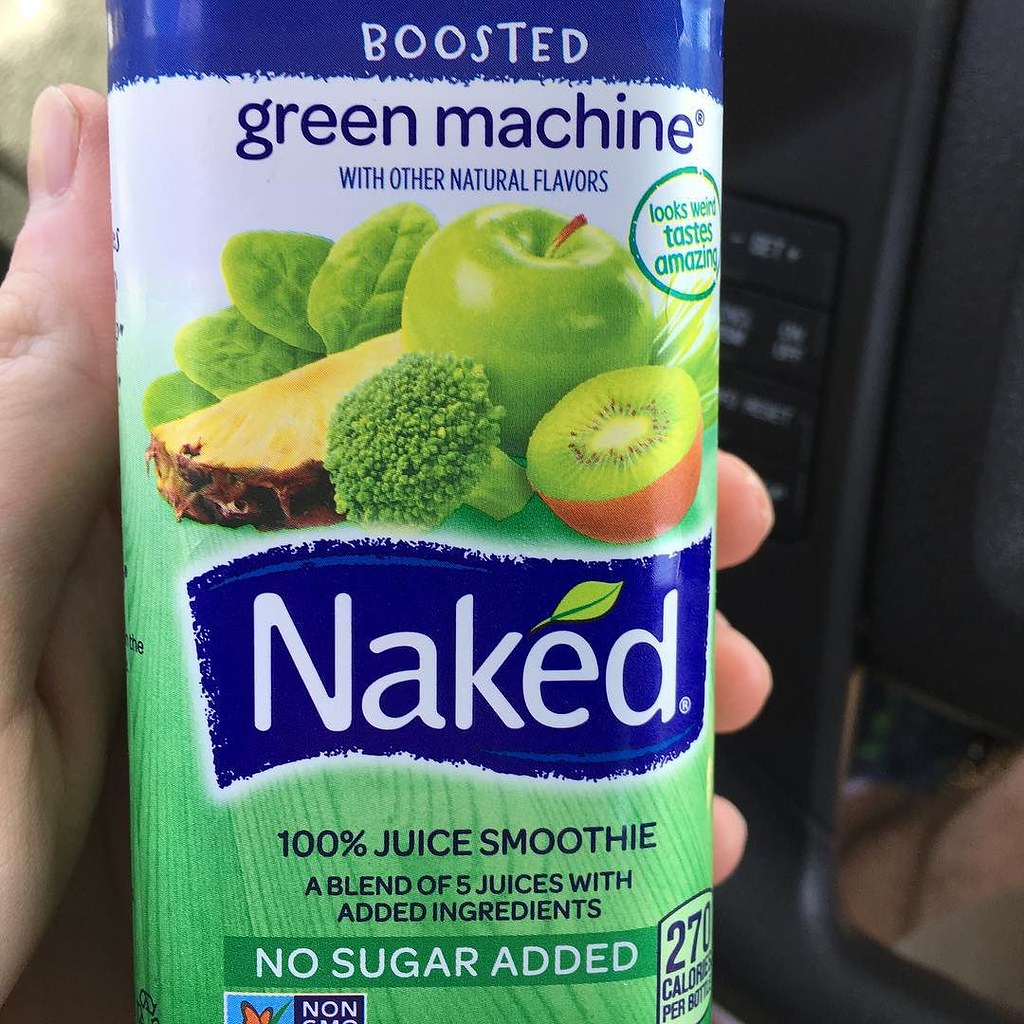In this image, a person is holding up a drink container labeled "Boosted Green Machine." The container boasts a vibrant design, featuring a green background with the word "Naked" prominently displayed against a blue backdrop. Above the brand name, there are colorful illustrations of various fruits and vegetables, including a green apple, broccoli, kiwi, pineapple, and what appears to be spinach. The label also highlights that the drink is a "100% juice smoothie," made from a blend of five juices with added ingredients, and reassures consumers with the note "no sugar added." The nutritional information indicates that the beverage contains 270 calories. The setting of the photo seems to be inside a car, as part of the dashboard is visible on the right side of the image.